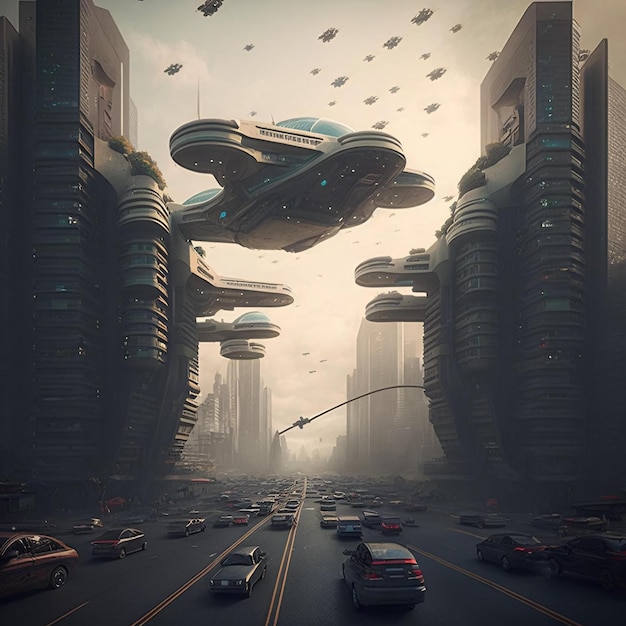This digital artwork portrays a sprawling futuristic cityscape dominated by towering skyscrapers and a massive, multi-lane highway teeming with traffic. The highway, consisting of at least ten lanes with cars in both directions, stretches across the bottom of the image, suggesting a bustling, densely populated metropolis. Flanking the highway on either side are immense, dark-colored skyscrapers, some of which boast verdant balconies, adding a touch of greenery to the urban environment. The impressive scale of the buildings continues into the background, where more high-rises punctuate the skyline.

Hovering in the sky, close to the ground and centrally positioned, is an intricate hovercraft, a hallmark of the futuristic theme. In the hazy, beige-tinged atmosphere above, additional flying vehicles, resembling robotic spaceships or alien shuttles, are scattered throughout the sky, bringing an air of advanced technology and possibly interstellar activity. The image has a cinematic quality, with sharp details in the foreground and a gradual, foggy blur as the perspective recedes, enhancing the sense of depth and the city’s vastness. The overall mood is dark and somewhat dystopian, suggesting a complex, perhaps chaotic future world.